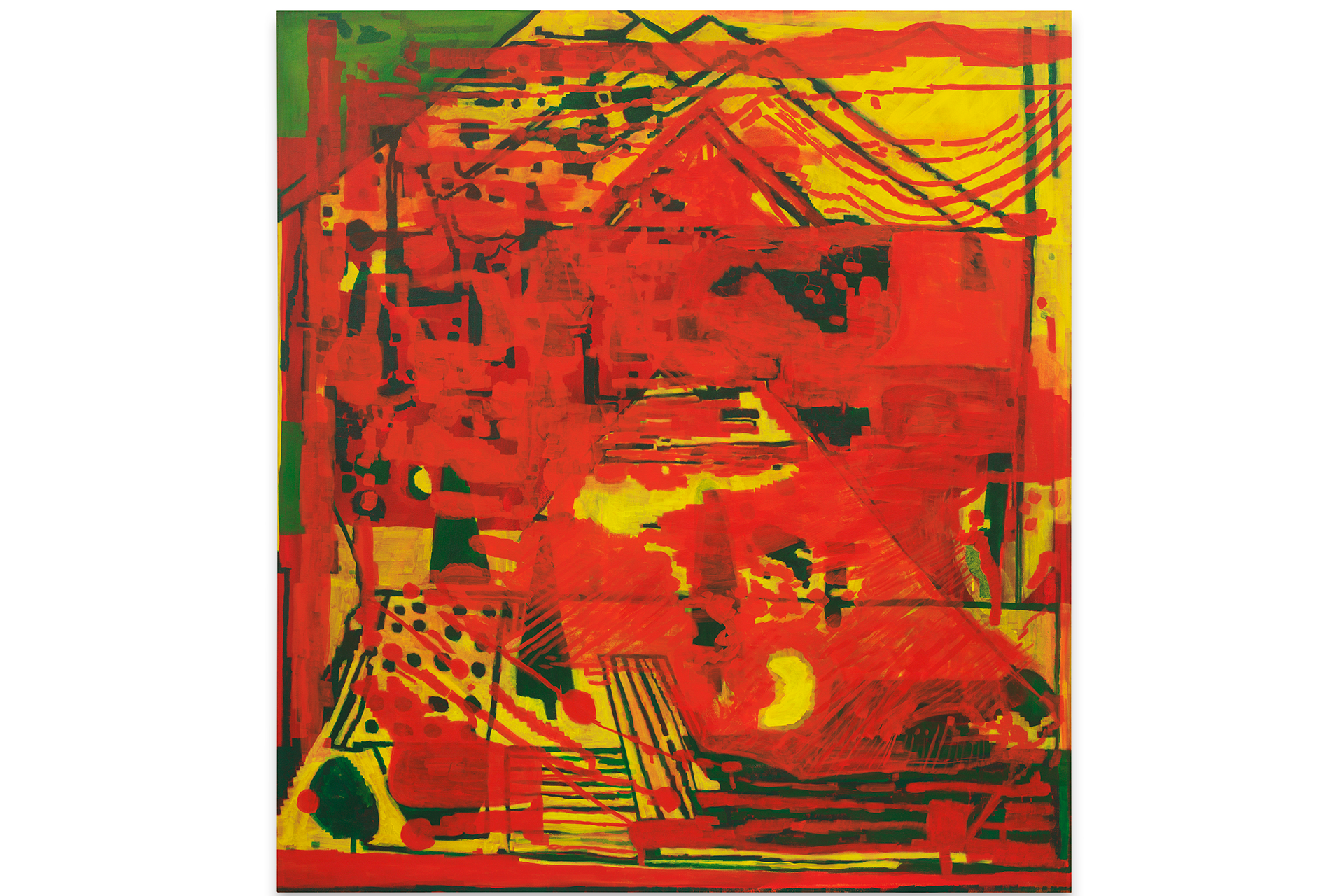This abstract artwork features a tumultuous composition dominated by vibrant hues of bright red, mustard yellow, grass green, and darker green. At the top of the painting, numerous overlapping pyramid shapes blend into a cascade of red streaks that permeate the entire scene, creating an almost chaotic texture. Central to the piece, a prominent yellow pyramid, partially obscured by the red streaks, emerges subtly from the vibrant background. The painting has a predominantly yellow background interspersed with dark green outlines forming various indistinct shapes and shadings. A notable section at the lower left captures attention with a rectangle dotted in black, layered with yellow and accentuated by additional red lines. Scattered throughout the artwork are irregular shapes, squares, and occasional green dots, adding to the complexity. The overall effect is a mesmerizing amalgamation of abstract forms, flowing brush strokes, and random paint dribbles, making it a striking example of abstract expressionism.